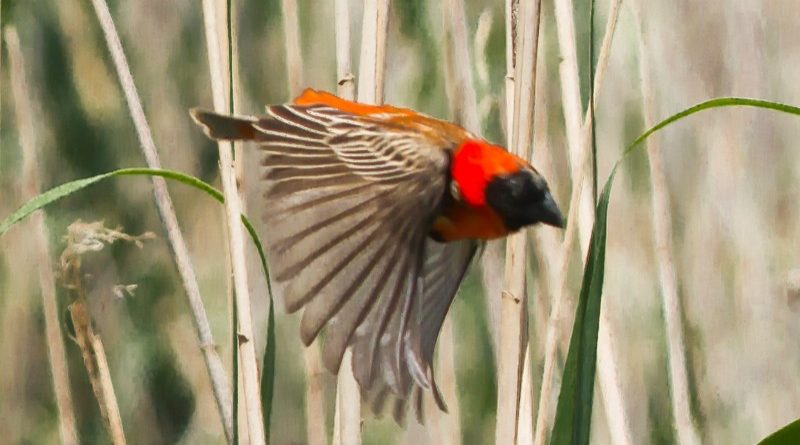The image depicts a bird in mid-flight within a marshy or grassy area. The bird, captured in a side view, is flying toward the right with its wings down, showcasing an impressive array of individual feathers. The bird has a distinctive black head and beak, with a striking red patch on its forehead. Its eyes blend into the black head, making them less distinguishable. The top part of the bird's body displays hues of brown, while the tail is gray. Its wings, appearing somewhat translucent, are gray with white lines and hints of off-white, orange, and brown. The backdrop features light gray branches and various vegetation suggestive of tall, dried grasses or cat-tails. Additionally, a few green grass tendrils are noticeable, contributing to the natural setting. The entire scene focuses on this elegant bird, highlighting the intricate details of its plumage and the serene environment through which it soars.